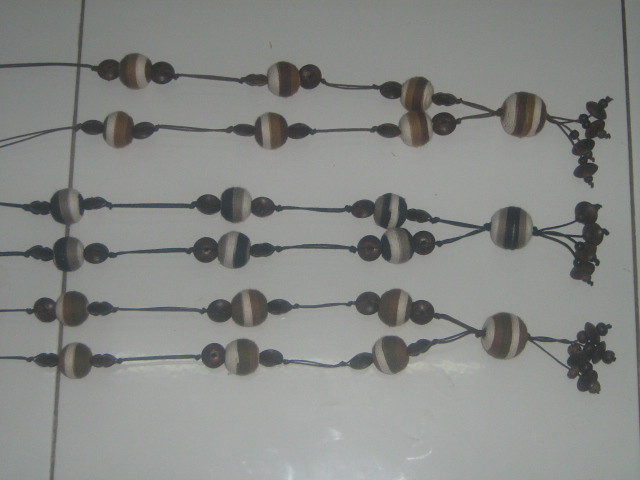In the color photograph, we look down onto a white surface where three bead necklaces are meticulously arranged side by side. Each necklace features a deliberate design pattern: evenly spaced sets of three beads anchored on a string or rope cord. The center of each set boasts a larger, approximately one-inch diameter bead with characteristic white stripes, flanked by two smaller round beads. This triad pattern repeats uniformly along the length of all three necklaces. 

At the far right of the image, all three necklaces converge at a single larger pendant. This pendant is an intricately patterned, round bead displaying alternating stripes of light brown, tan, black, and white. Extending from the base of this central pendant are multiple black strands adorned with smaller brown beads, each about a quarter inch in diameter. The beads lie across a white background, which might be a table or some other plain surface, and the image is slightly dark but remains in clear focus. There are no words or text present within the frame.